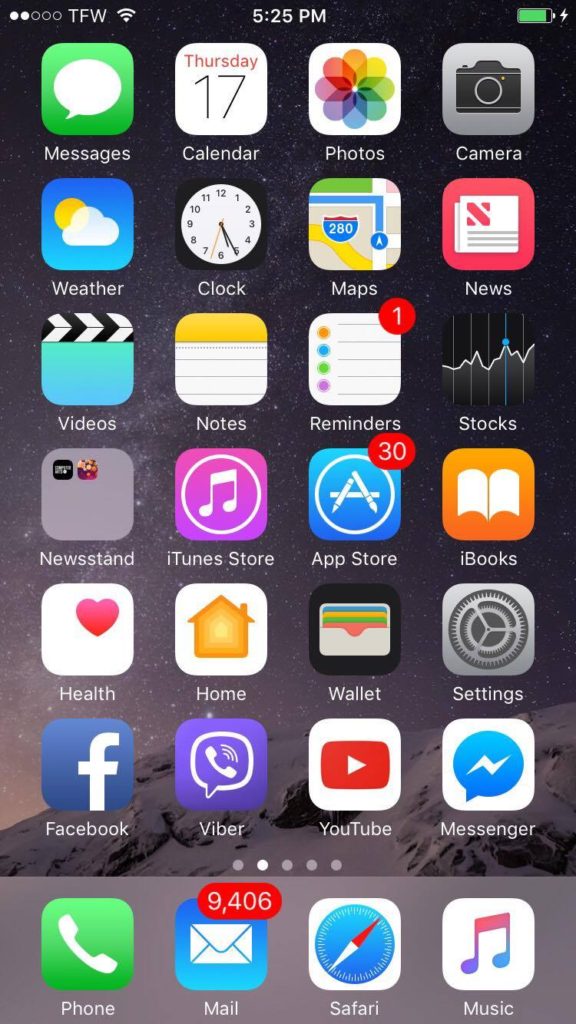This image captures the screen of someone's cell phone, displaying an interface against a background that resembles a wintry night sky. The backdrop predominantly features a black expanse sprinkled with white specks and faint luminescence, evoking the impression of a snowy landscape under a starlit sky. Silhouettes of snow-capped hills or mountains are faintly discernible in the distance, enhancing the wintry atmosphere.

At the top of the screen, five status dots are visible, with two filled in and three hollow. The acronym "TFW" is displayed beside the connectivity indicator. The time, "5:25 PM," is prominently shown at the top center of the screen. In the upper-right corner, the battery icon, filled with green to signify charging, is also present.

The app icons are systematically arranged in a grid pattern, with four icons per row and seven rows in total. The primary app icons include Messages, Calendar, Photos, and Camera, followed in subsequent rows by Weather, Clock, Maps, News, Videos, Notes, Reminders, and Stocks. At the bottom of the screen, a rectangular dock houses four additional frequently-used app icons, completing the organized and functional layout of the home screen.